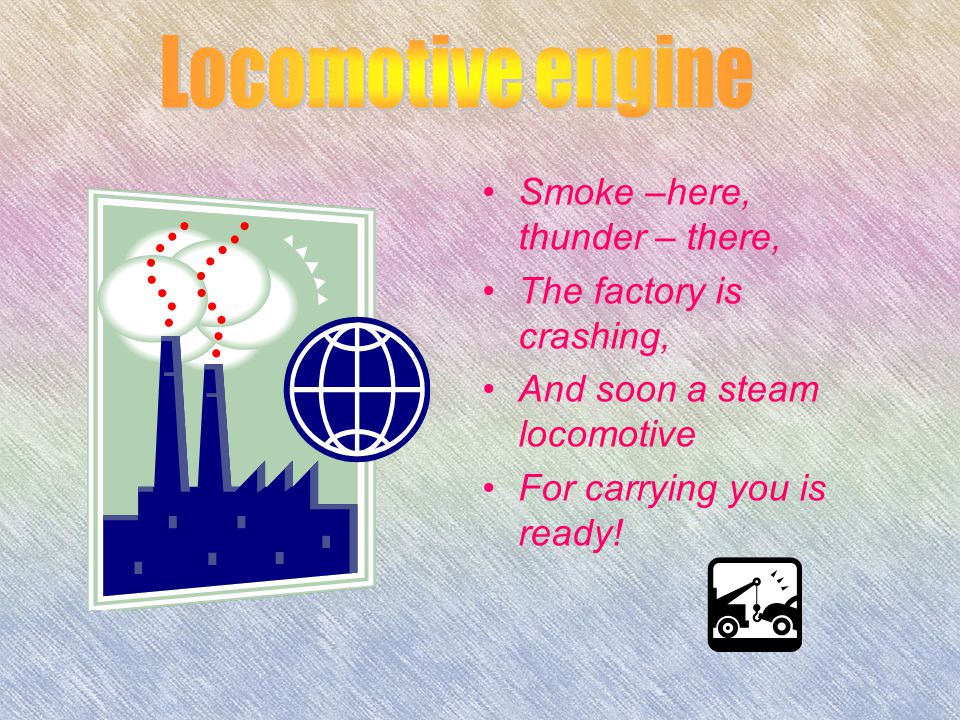The image is an informational slide designed for a presentation, featuring a colorful, multi-hued background that transitions from blue at the bottom to green, purple, and finally orange at the top, interspersed with various white dashes. Prominently displayed at the top of the slide is gradient orange text that reads "Locomotive Engine." Beneath this are multiple lines of pink text stating, "Smoke here, thunder there. The factory is crashing, and soon a steam locomotive for carrying you is ready."

On the left side of the slide, there's a clip art illustration depicting a blue factory with white smoke clouds emanating from two chimneys, underlaid with red dots. A globe with blue and white meridian lines sits atop this factory depiction. In the lower right corner, there's another piece of clip art showing a black tow truck towing a car against a white background. The overall setting suggests a PowerPoint presentation, likely used within an educational context. The slide is visually engaging with its bold color scheme and eclectic mixture of imagery and text, aimed at capturing the viewer's attention.